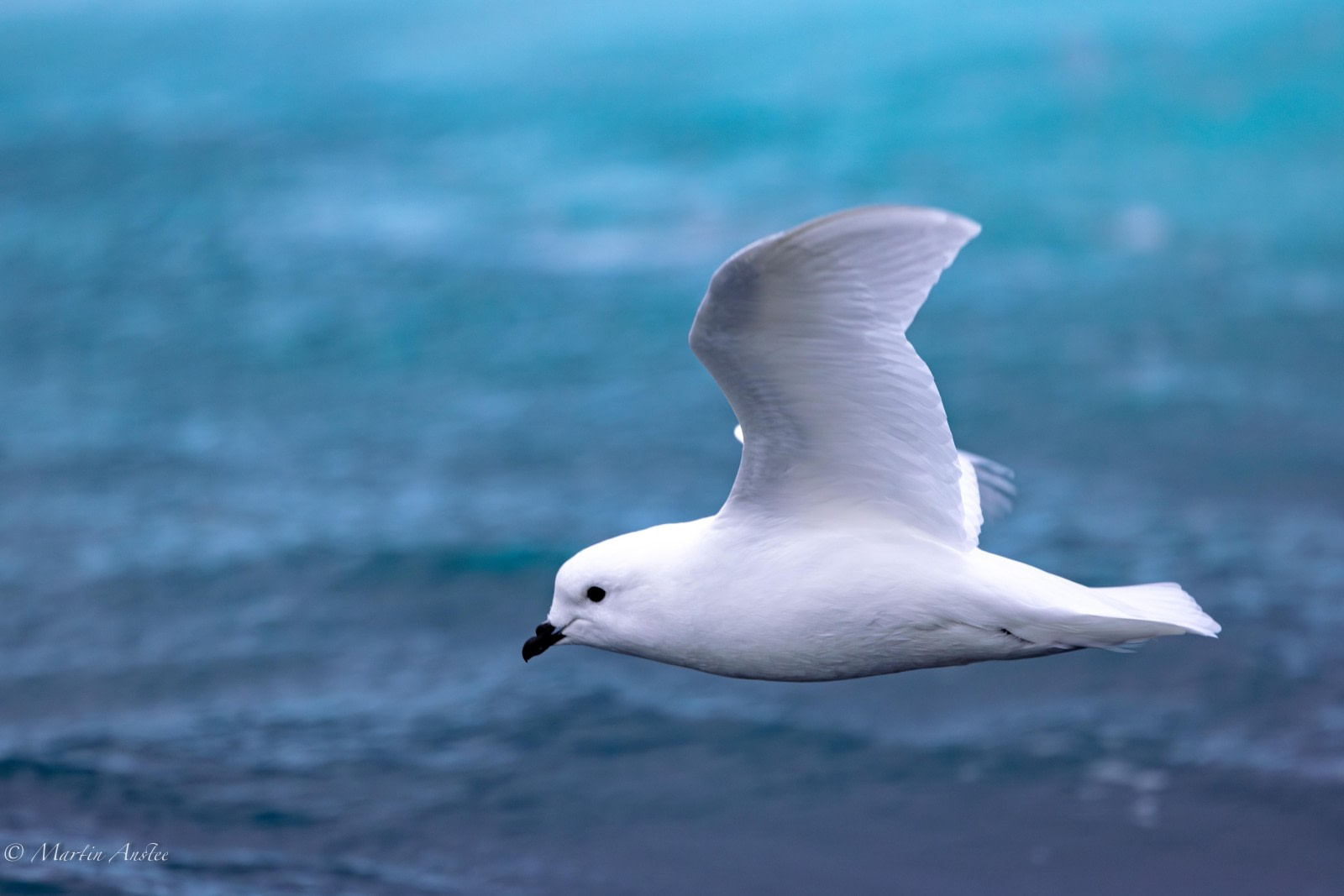A graceful medium-sized bird, characterized by its white plumage, black beak, and black eyes, soars effortlessly over the ocean. It appears to be a species that dwells on seaside cliffs, caught mid-flight with its wings elegantly raised and its feet tucked in. The background, though blurred, reveals a stunning gradient of the ocean's colors, transitioning from darker shades at the bottom to lighter, enchanting hues of turquoise mixed with hints of purple at the top. This variation of colors adds to the overall beauty of the scene. In the bottom left corner, the photographer's credit, "Martin Oster," is subtly inscribed in white text, underscoring the artistry behind this captivating image.